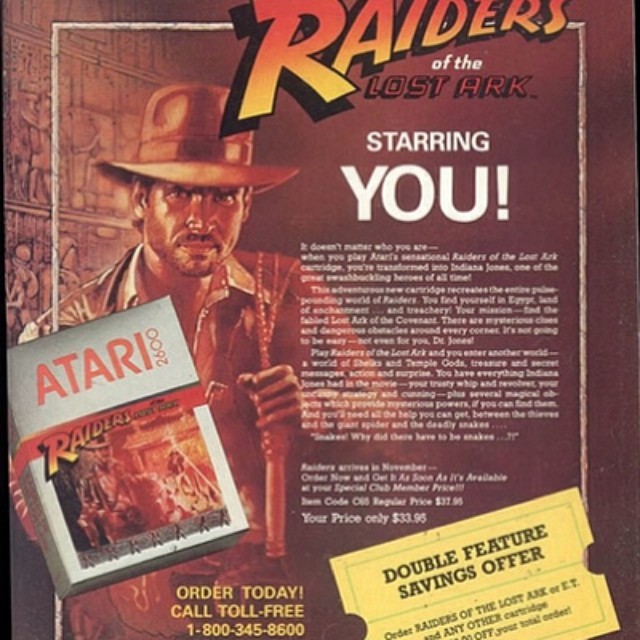This image showcases a nostalgic advertisement for the classic video game, "Raiders of the Lost Ark," designed for the Atari 2600. In the top-right corner, the game title "Raiders of the Lost Ark" is prominently displayed, with "Raiders" written in striking red and orange gradient letters outlined in black, while "Lost Ark" is in white. Adjacent to the title is the phrase "Starry New," also in large white letters. 

Beneath this, a block of promotional writing spans multiple paragraphs, but the low resolution renders the text unreadable. Further down, more detailed information is present, with the only decipherable detail stating, "your price, only $33.95." 

The lower section of the ad features a yellow movie theater-style ticket with semi-circular cutouts at both ends, announcing a "Double feature savings offer." It invites customers to order "Raiders of the Lost Ark or E.T." alongside any other cartridge, though the bottom part of the offer details is cutoff and unreadable. The ad encourages immediate action with the instruction, "Order today. Call toll-free 1-800-345-8600."

In the foreground, the iconic silver cartridge of the game is depicted with "Atari 2600" in bold red letters. The game's cover showcases an adventurer in a cowboy hat wielding a whip, visually echoing the character of Indiana Jones from "Raiders of the Lost Ark." The same figure is mirrored on the silver game box. Behind the forefront elements, a gradient orange background further highlights the adventurous theme of the game.